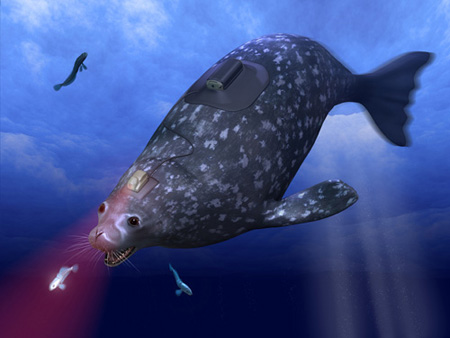In this underwater digital art image, a sizable, dark gray seal with white spots and a distinctive white mark around its eye, resembling the number 5, is depicted swimming toward a small, white fish, with its mouth wide open as though about to eat it. The scene is set near the water’s surface, with sunlight streaming down into the water, creating a radiant atmosphere. There are a few minor fish swimming around, adding to the underwater ambiance. The focal point is the seal, which is equipped with two large, centrally placed laser attachments: one on its back and another on its head. The device on its head emits a red laser beam, highlighting the fish it is targeting. The imagery includes a backdrop of white clouds visible through the surface and a ray of light piercing down into the ocean, enhancing the surreal and possibly fabricated nature of the scene.